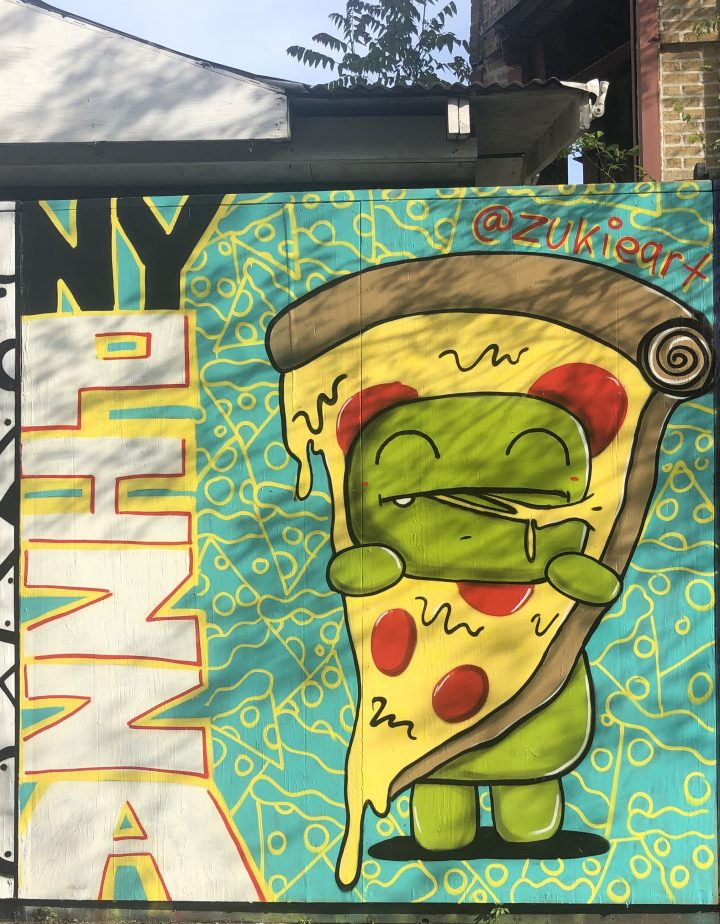This image depicts a close-up of a vibrant mural on the side of a building, featuring a striking blue background adorned with repeatedly drawn yellow pizza slices. Dominating the mural is a large, cartoonish green dinosaur whimsically dressed in a pepperoni pizza costume, complete with a brown crust, yellow cheese, and red pepperoni slices. The dinosaur's head pokes through the pizza slice, and its simple eyes are shown as curves while its mouth is open. The dino's hands, clenched into fists, are visible around the edges of the pizza suit. At the top left corner of the mural, "NY" is emblazoned in big black letters outlined in yellow, and just below it, the word "PIZZA" is vividly displayed in large white letters, enhanced with yellow and red outlining. To the top right corner, the artist's handle "@zukiart" is inscribed above another slice of pizza, adding a signature touch to this lively and creative piece.